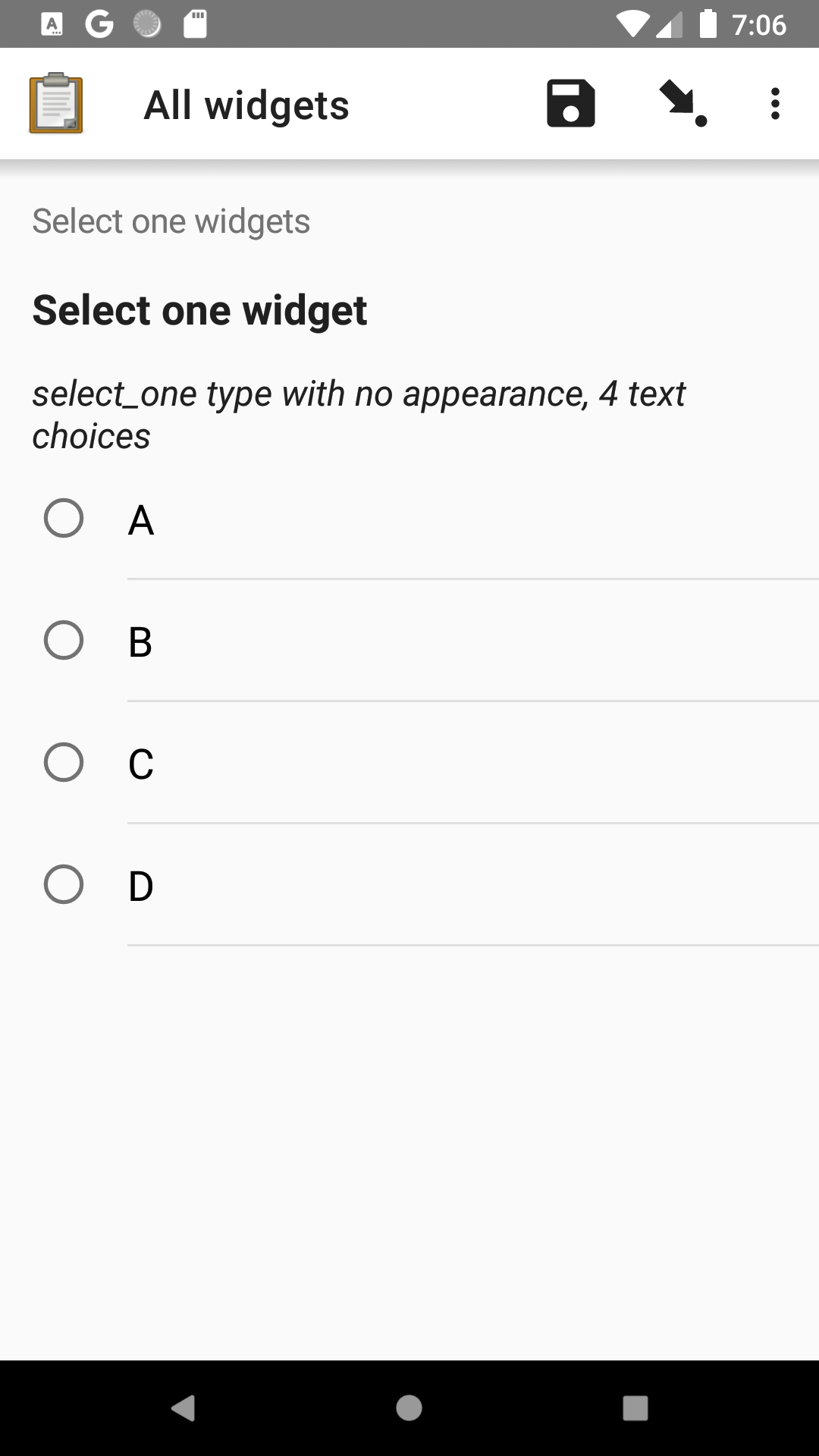In the upper portion of the image, there is a dark gray bar featuring several icons. On the left side of this bar is the Google "G" logo, while the right side displays a Wi-Fi symbol with half the signal bars, a fully charged battery icon, and the time, which shows 7:06. Directly below this bar is a white area; on the left side of this section is a clipboard icon with a piece of paper, alongside the text "All Widgets." To the right of this text is a disc symbol, followed by a black circle with a black arrow pointing towards it. Additionally, there is a vertical ellipsis to the far right. 

Below this header section is a gray background with the phrase "Select One Widgets" in gray text at the center. Underneath this, in bold black text, is the heading "Select One Widget." Beneath this heading, in black italic text, it reads: "Select_one_type with no appearance, four text choices." Following this, there are four circles arranged vertically, each with a light gray interior and a black border, labeled A, B, C, and D respectively. Adjacent to each circle is a light horizontal gray line.